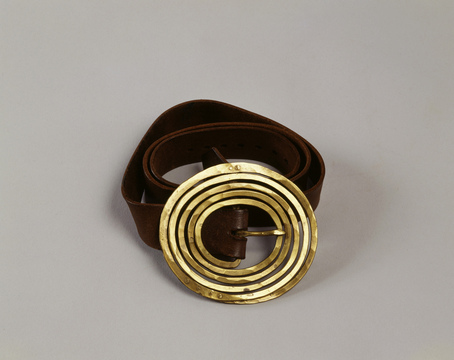The image features a brown leather belt, artfully coiled in an irregular spiral on a solid white surface, with the coil forming a clockwise direction. The belt lies flat on its thin edges, giving the appearance of a delicate, contemporary art piece. Dominating the foreground is a unique, gold-colored belt buckle, characterized by its striking circular design. The buckle consists of five concentric rings, each slightly uneven, suggesting a handcrafted touch. The buckle radiates an intricate gold spiral pattern, ending in a small pin, matching in color, designed to secure the belt through its eye holes. Soft shadows cast across the scene hint at a light source positioned behind the camera. The belt is meticulously centered within the frame, emphasizing its artistic and detailed presentation.